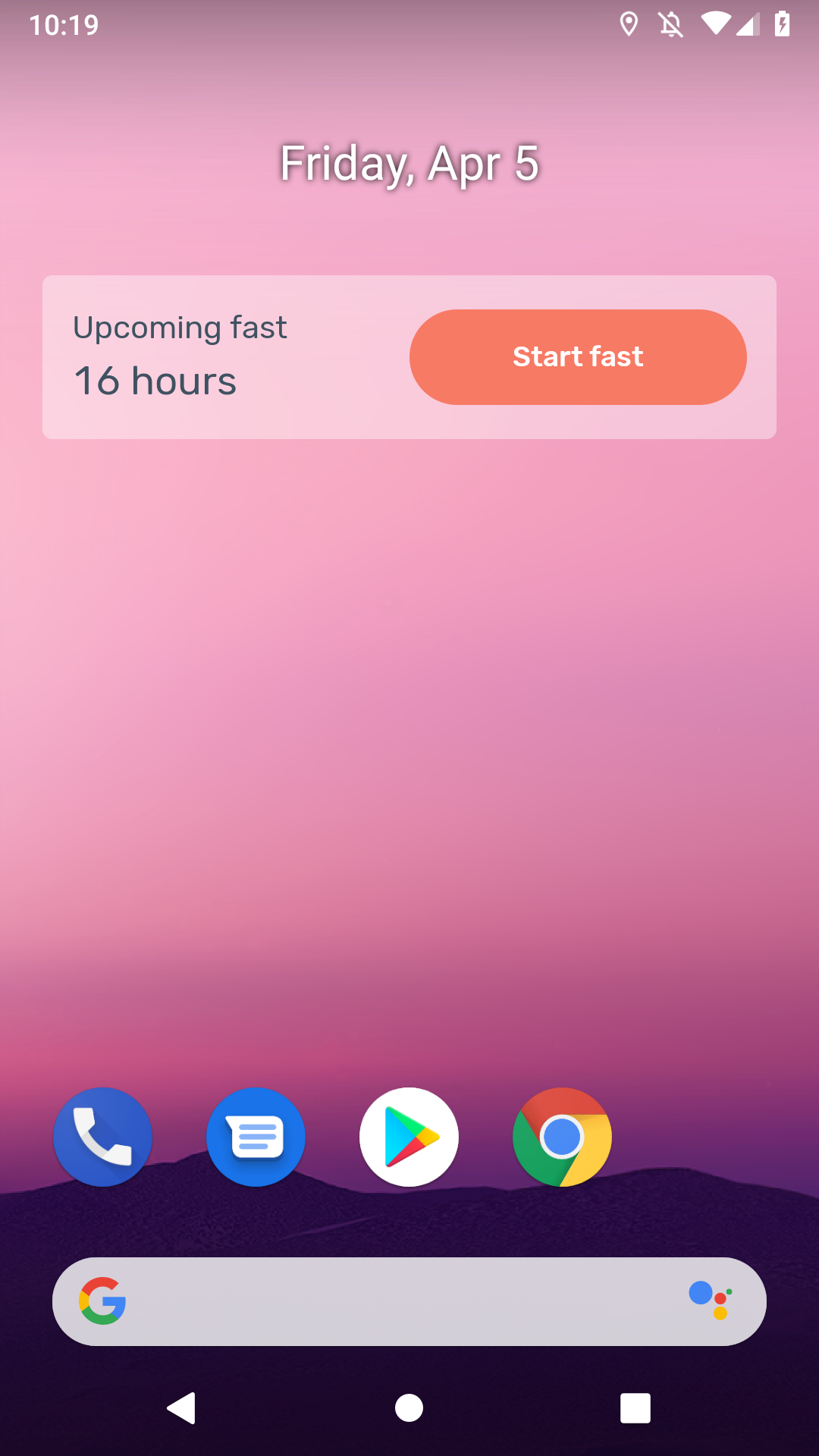The image depicts a screenshot of a smartphone's homepage. At the top of the screen, the date and day, "Friday, April 5," are displayed in white text. Beneath the date, there is a white notification box that reads, "Upcoming Fast, 16 hours," on the left side. Positioned to the right of this notification is an orange, pill-shaped button labeled "Start Fast."

Further down the screen, at the bottom, are four app icons arranged horizontally: a green "Call" icon, a blue "Messaging App" icon, the "Google Play Store" icon, and the "Google Chrome" icon. Below these icons, the Google search bar is prominently positioned, featuring the Google "G" logo on the left side.

The background imagery of the phone screen features a serene landscape, with a pink gradient sky that transitions to purple as it approaches the horizon. The lower portion of the background reveals a silhouette of purple mountains, enhancing the tranquil aesthetic of the device's interface.